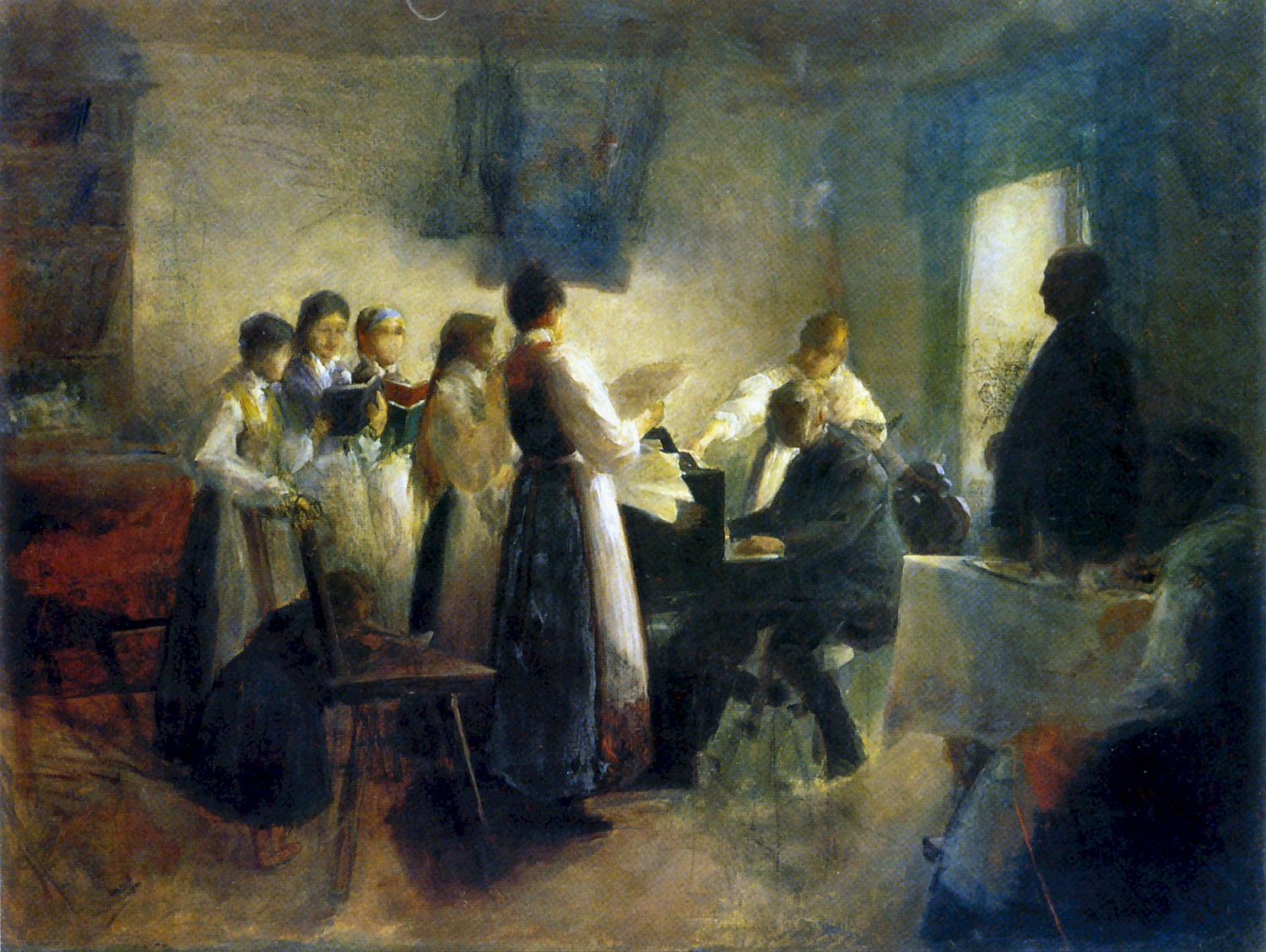The image depicts an interior scene from colonial times, rendered in a slightly impressionistic style using oil pastels. Central to the composition is a person seated at either a piano or harpsichord, dressed in a blue suit, playing as several individuals stand around. The scene is set in a large room with plastered walls, displaying various shades of white and blue that reflect different light sources. 

In the foreground, a woman wearing a colonially styled dress with a white apron stands to the far right, possibly holding another piece of fabric. The group surrounding the seated figure consists of both men and women, many with dark hair pulled back into buns or braids. One figure, distinguished by a tall stature and a braid, stands near a window adorned with blue drapes on the upper right part of the painting. 

The background features a mix of dark and lighter blue splotches, creating a dynamic and textured effect, contributing to the overall impressionistic aesthetic. Near the center-right portion, there's a table draped with a white tablecloth, possibly supporting a vase or similar object. The composition also includes a white door in the background and a person leaning against it. One prominent character in brown smock and white shirt is pointing, drawing attention to the musical performance or another focal point within the scene. The figures lack intricate facial details, adding to the impressionistic quality of the artwork.